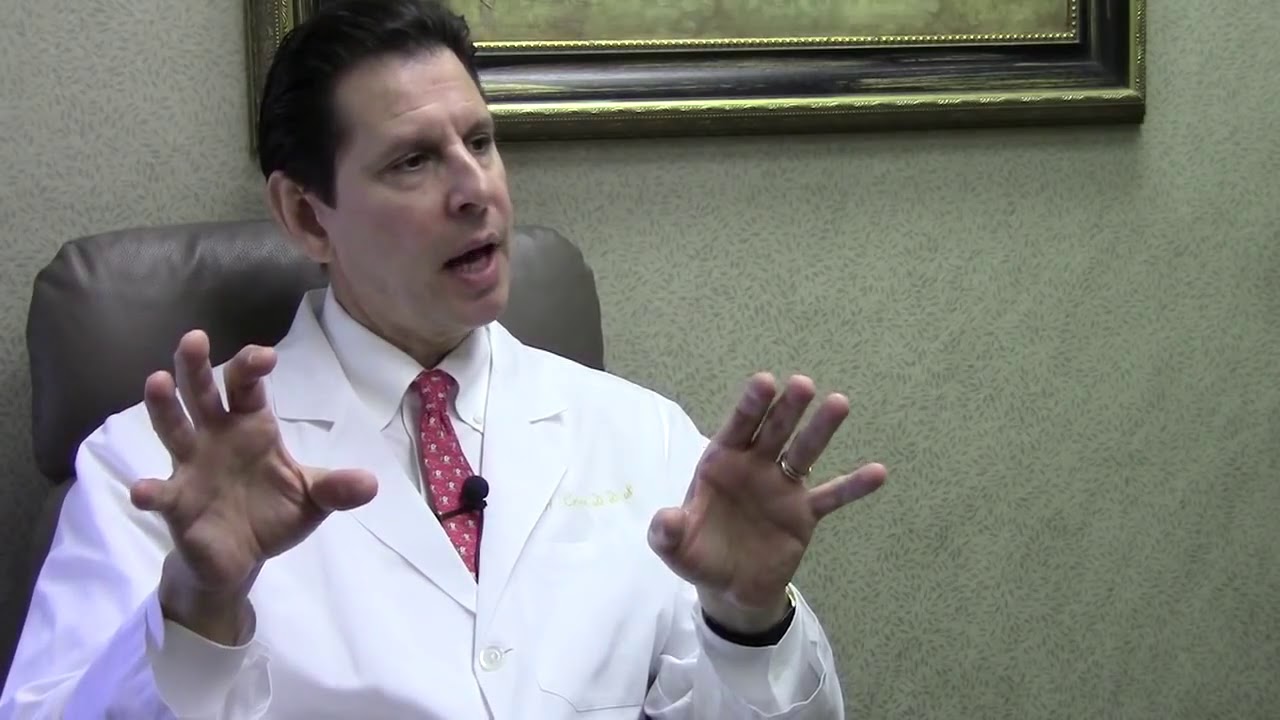In this horizontally oriented image, a middle-aged man, presumably a doctor, is seated in a brown leather chair. He has short brunette hair and is adorned in a white, buttoned-up lab coat over a white dress shirt, complemented by a red tie that has a small microphone attached to it. He appears to be engaged in a conversation or interview, captured mid-speech with his mouth open and his head turned to the right. His hands, featuring a wedding ring on his left fourth finger, are raised to shoulder height with fingers spread apart, as if making a descriptive gesture. The background showcases beige walls with a greenish tint, highlighted by the bottom edging of a gold-framed picture hanging behind him. His detailed attire, expressive posture, and the subtle elements of the setting collectively convey a professional setting where he might be explaining a situation or problem.